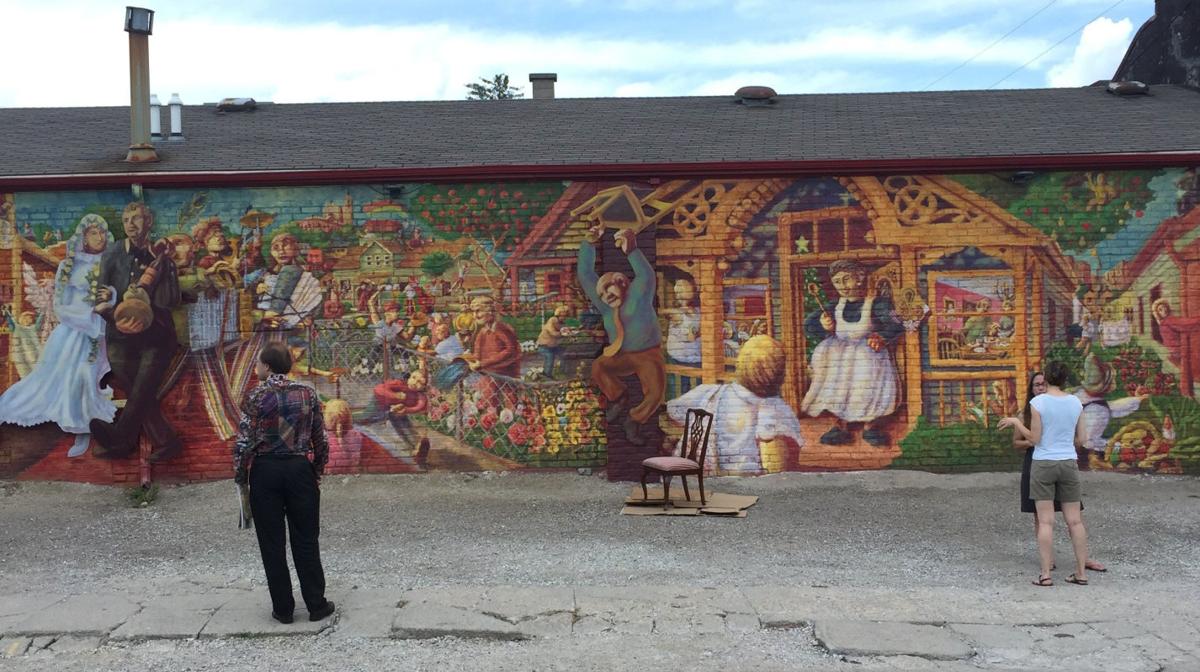This daytime photograph captures a vibrant mural painted on the side of a brick building, becoming the focal point as it stretches from the center left to the center right of the image. The mural vividly portrays various life events: on the far left, a scene of a marriage with a man in a uniform accompanying a woman in a bride’s dress, surrounded by celebratory people. Toward the center, there's a poignant depiction of a man upset, breaking a chair, and nearby, a pair of grandparents—one jubilant, the other appearing enraged. To the right, a woman in an apron, holding a wooden spoon, stands in the doorway of a small, colorful cottage, possibly overseeing the scene. The surrounding landscape includes green buildings with brown rooftops and fruit-laden bushes, adding to the mural's depiction of a charming small town.

The sidewalk in front of the mural is made of cracked cement and is bordered by a gravel courtyard, clearly in disrepair. An empty chair rests on some flat cardboard at the center of the image. A group of people is looking at the mural; among them are two women engaging in conversation on the right, a man in a colorful spotted shirt with a balding head intently observing the mural, and a couple standing close, holding hands. The man is wearing long black pants and a long-sleeved shirt, while the woman is clad in a light blue shirt paired with dark green or gray shorts. These figures add a dynamic realism to the artwork.